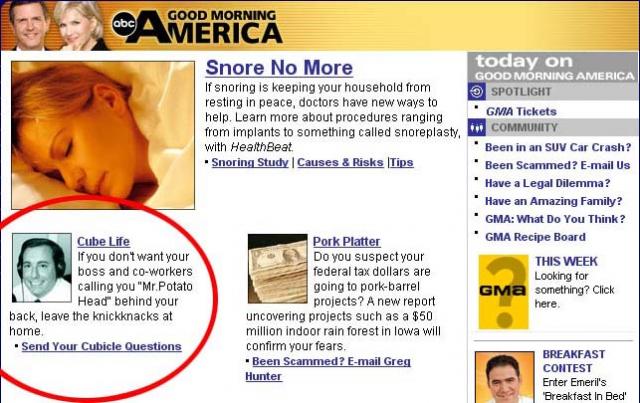The image is a screenshot of an old website for "Good Morning America," identifiable by the "Good Morning America" logo in the upper left corner. The webpage displays several articles and features. On the left side, a list of articles includes one highlighted in red titled "Cube Life," advising against bringing personal knickknacks to work to avoid being teased. Another article mentioned is "Snore No More," which discusses medical treatments for snoring, including implants and a procedure called snorplasty. On the right side of the image, there's a sidebar labeled "Today on Good Morning America" with a schedule of upcoming shows and additional links and features, including spotlight and community segments. The background suggests it is an older design, emphasizing the website layout typical of earlier internet eras.